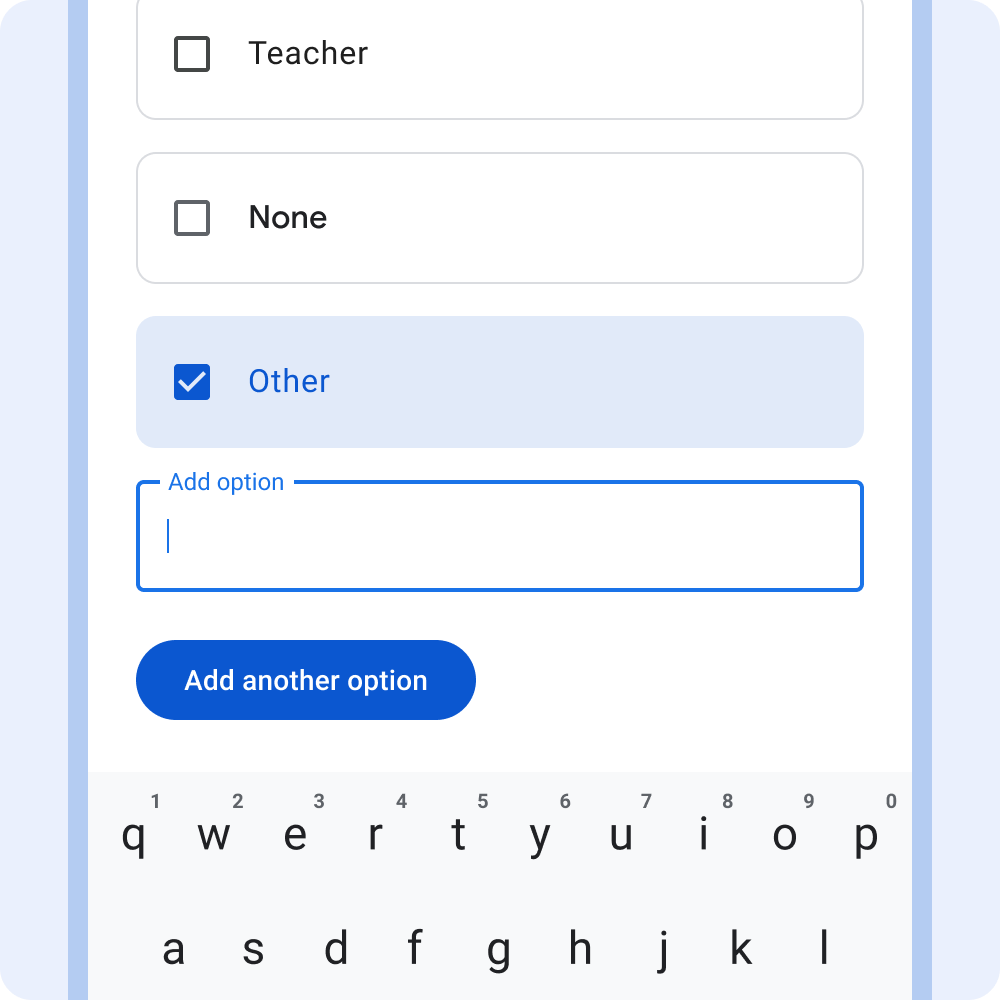This image is a screenshot from a mobile device. The borders of the image are a light grayish-blue color, with a darker blue bar at the top. The left and right edges of the image also have these colors. In the center section, there is a white background.

At the top of the white portion, there are three main rectangular boxes. To the left of each box is a smaller, dark grayish-black square. Each of these smaller squares has a label to its right. The labels, starting from the top, are as follows: 
1. "Teacher"
2. "None"
3. "Other"

The "Other" option is marked with a check mark. Below these three options, there is a box labeled "Add option." Directly beneath this label, there is an interactable button also labeled "Add option." Continuing downwards, the bottom part of the image shows the top half of a keyboard.